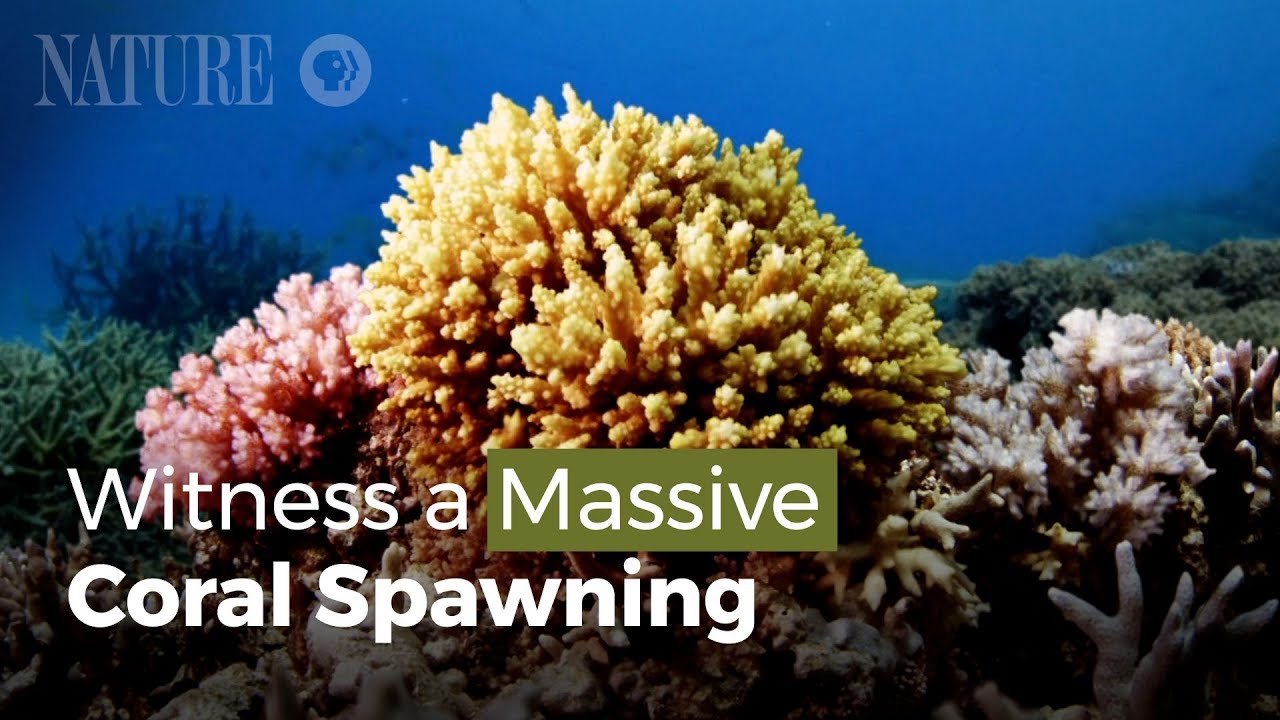This vibrant underwater scene captured at the bottom of the ocean showcases a diverse coral reef teeming with life. At the top left, the image includes the text "NATURE" alongside the PBS logo, featuring a stylized profile of a human face. The background is characterized by dark blue ocean water. Dominating the center is a large yellow coral, reminiscent of caramel popcorn, bordered on the left by a pink coral and on the right by a white coral. The scene is further enriched by green coral and various rock structures. In the bottom left corner, the text "witness a massive coral spawning" is prominently displayed, with "massive" highlighted within an olive green rectangle, and the rest of the text in white. This image embodies the vibrant marine biodiversity expected in a PBS Nature documentary.